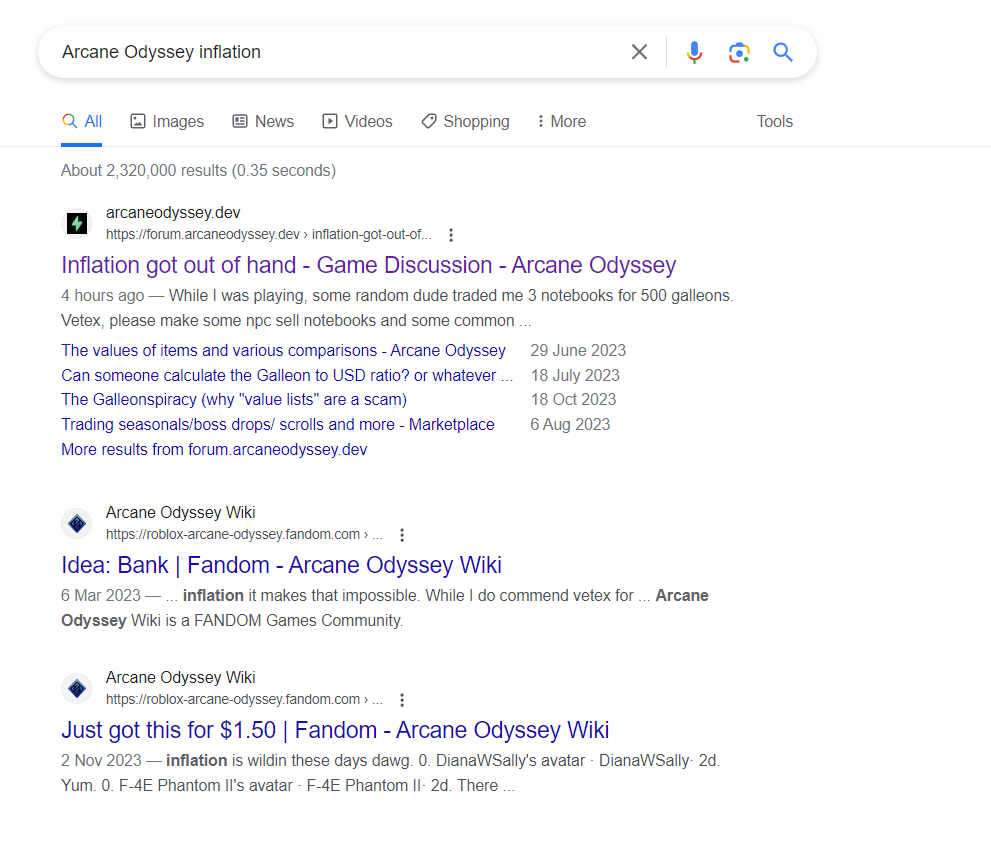The image depicts a Google search results page for the query "Arcane Odyssey inflation." At the top of the page, the search bar is prominently displayed with the query text. The results page includes standard tabs such as All, Images, News, Videos, and Shopping, with the "All" tab being highlighted in blue. The search yielded approximately 2,320,000 results in 30.35 seconds.

The visible search results focus on discussions and concerns about inflation within the Arcane Odyssey game. Key highlights include a forum post about a player trading three notebooks for 500 galleons, another user's plea to developer Velltex to have NPCs sell notebooks to stabilize the economy, and comparisons of item values within the game. Additionally, there are requests for calculations of the in-game currency's value relative to USD, debates on the legitimacy of value lists, and various trading posts for seasonal items, boss drops, and scrolls. 

The results seem to be drawn from various forums and wikis dedicated to Arcane Odyssey, including forum.arcaneodyssey.dev and the Arcane Odyssey Wiki.